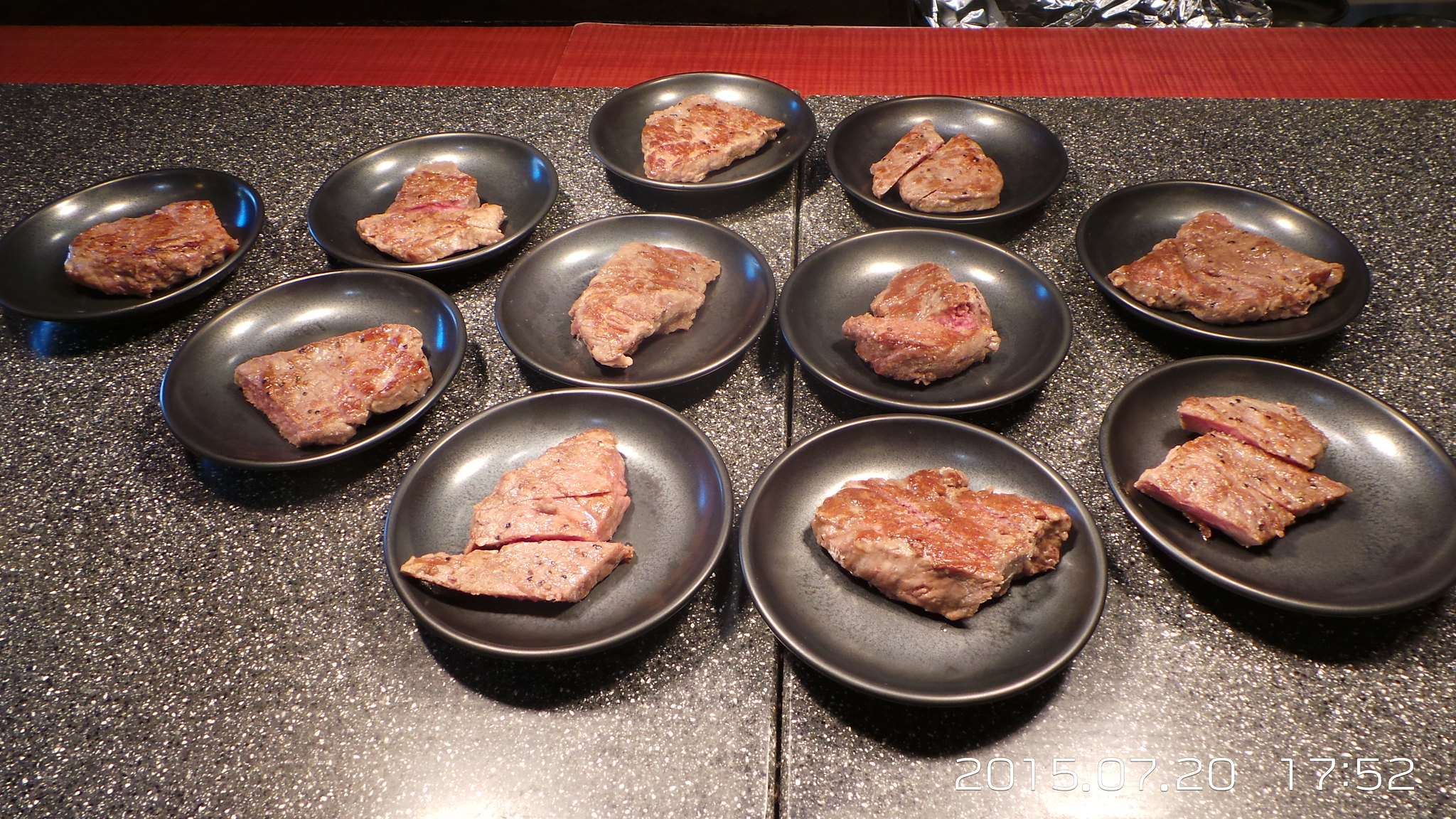A detailed image taken on July 20, 2015, at 5:52 PM, displays a matte black table with specks of white, dark black, and light brown across its surface. The table appears to be composed of two sections joined together, highlighted by a visible line running through its middle. Atop this table lie approximately ten cast iron pans, each containing steaks that are cooked to rare doneness. Some steaks are sliced into pieces while others remain whole. The table also features a red fabric element running along the top edge and a time-stamp noting the date and time of the photo. The surrounding ambiance hints at a stone or similar material finish, providing a reflective surface that adds to the visual detail of the setting.